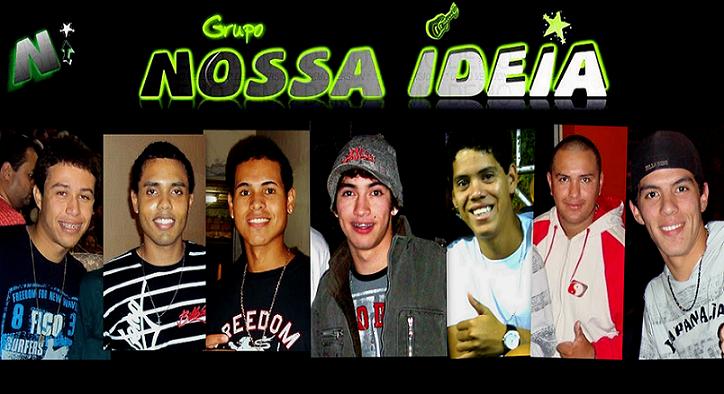The image is a long, black background poster for a band named "Grupo Nosa Idea." At the top, in neon green letters, the band's name is displayed with a small guitar for the dot of the "i" and a star above the uppercase "I." In the top left corner, there's an icon featuring letters "N" and "I" on a neon green background. The poster showcases seven young males, all smiling directly at the camera. Their portraits are separated but arranged in a line from left to right. 

The first member, with brown hair, is wearing a blue shirt and a silver chain. The second has similar brown hair and is dressed in a blue and white striped shirt with a silver chain. The third, with possibly brown or black hair, is sporting a shirt that says "Freedom" and is also wearing a silver chain. The fourth member, donning a gray hat, has dark hair and is clad in a gray overcoat over a gray or blue shirt with red writing. The fifth member has black hair, a watch, and a black and white shirt. The sixth member, who is nearly bald yet has dark hair, wears a red and white hoodie. The seventh individual, with a black hat and likely dark hair, is wearing a white and black shirt with the text "Yapana.ip," along with a silver chain.

Each member is dressed in modern attire, predominantly in a color scheme involving white, black, gray, and red. The imagery and layout suggest a young, vibrant boy band likely aimed at a youthful audience. Despite their separate portraits, their cohesive smiles and unified visual theme present them as a single collective group.